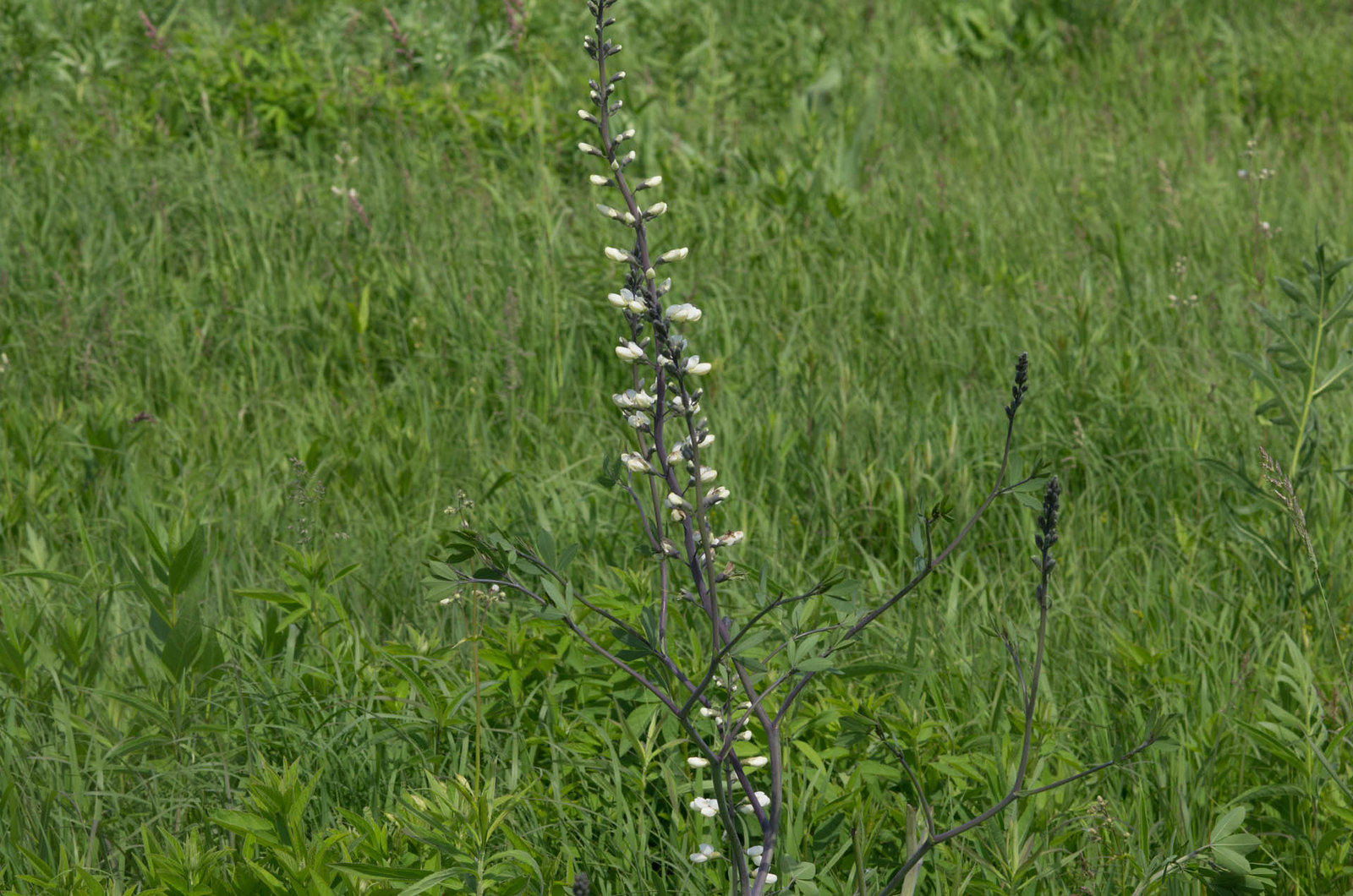This outdoor photograph captures a vibrant scene dominated by a rich green background of dense, tall grass, likely about a foot high, mixed with various weeds and wildflowers. The focal point of the image is a distinctive plant that stands taller than the surrounding greenery. This plant features slender, grayish-brown stems or branches that extend from the bottom center of the photo and converge near the top. Adorning these stems are numerous small, white flower buds, some of which display hints of green at their bases. These buds progress along the branches and increase in density towards the top, indicating they are in the early stages of blooming. The overall contrast between the verdant background and the striking, flower-laden stems creates a captivating and detailed nature scene.